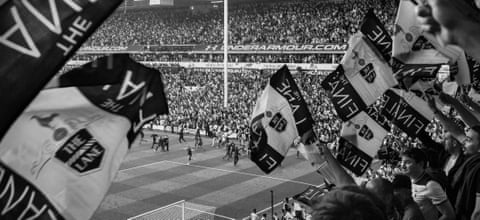The image is a black and white photograph of a soccer match, likely captured recently but stylized to appear vintage. In the foreground, there is a pristine, white soccer goal, and the meticulously cut field displays beautiful, proportional stripes in alternating shades of gray. The stadium is packed with thousands of excited spectators spread across three levels of stands, many of whom are waving flags and banners, although their text is mostly indecipherable except for one prominent sign that reads "The Lane" with an emblem featuring a bird perched on a ball. Another noticeable detail is the large Under Armour logo and "UnderArmour.com" printed on an awning, indicating sponsorship. This logo's clarity suggests the photo's recent origin. The sea of "The Lane" flags fluttering adds to the dynamic atmosphere, with some seemingly floating in mid-air. Players can be seen on the field, some captured mid-action, further energizing the scene.